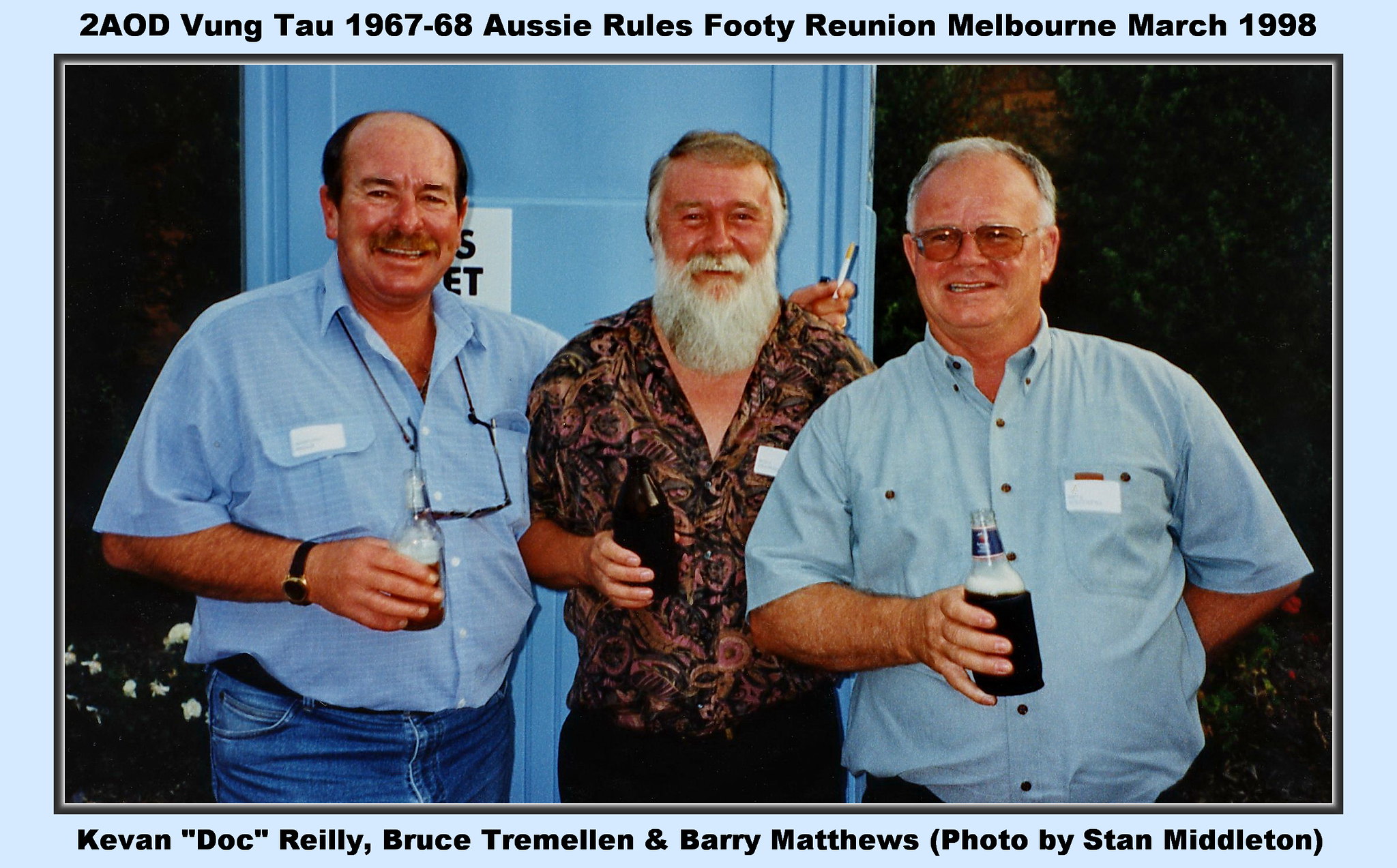The photograph captures a reunion moment of three older men, commemorating the 2AOD Vung Tau, 1967-68, Aussie Rules Footy Reunion in Melbourne, March 1998. The image is framed within a light blue border, which bears the aforementioned reunion details at the top, and the names "Kevin, Doc, Riley, Bruce Tremelin, and Barry Matthews" along with "Photo by Stan Middleton" at the bottom. 

From left to right: The first man sports a light blue collared shirt with the sleeves rolled up, blue jeans, and a black watch on his right wrist. He has balding hair and glasses hanging from a string around his neck, while he holds a cigarette behind the second man's head, adding a playful touch to the scene. 

The middle man stands out with his full white beard and light-colored hair. He wears a paisley shirt with a few buttons casually undone and black pants. 

The third man, positioned on the right, is also balding with gray hair and is wearing glasses. He dons a blue button-down shirt and black pants while holding a beer bottle. 

All three men are holding beer bottles and appear to be in good spirits, enjoying the moment captured by the camera.